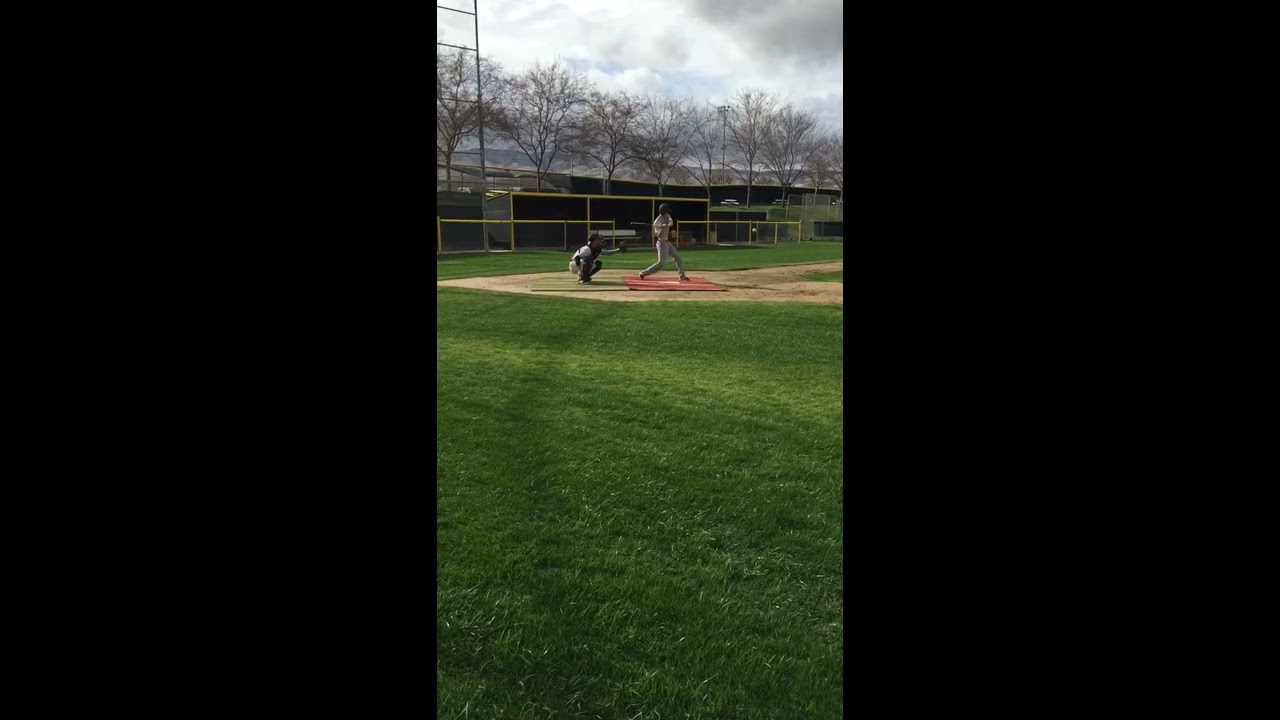In this detailed photograph of a baseball game, the image is centered between two large black rectangles, creating a striking contrast. At the heart of the image, the grass appears lush and impeccably maintained, stretching around the well-manicured baseball diamond. The focus is on the batter and the catcher, both small but clearly visible at home plate—a red dirt square with a pristine white base. The batter is captured mid-swing, the bat poised behind him, while the catcher crouches on his knees, mitt ready to catch the ball. In the background, a typical baseball fence about four feet high borders the field, with trees just beyond it, their leafless branches indicating a spring or fall game. The sky overhead is a mix of gray clouds with occasional glimpses of blue, and no spectators are visible. The overall scene exudes a peaceful, well-kept atmosphere, dominated by the vibrant green grass in the foreground.